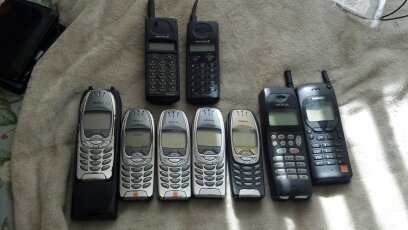The photograph showcases nine vintage mobile phones arranged on a gray towel, possibly resting on a floor or tabletop. The composition features two rows: the top row contains two black phones, while the bottom row includes seven phones, predominantly silver and black in color. Four of the phones appear to be classic Nokia models, with buttons and small screens, while the remaining five are even older, bulkier models, suggesting an earlier run of Nokia phones. There is notable natural light spilling into the frame from a window, illuminating the bottom right edge and casting a shadow over the right-hand side. One phone in the bottom row appears to be sitting on a case or object, contributing to the subtle variation in their alignment. A glass object, possibly a table, is also barely visible in the top right corner of the photograph.